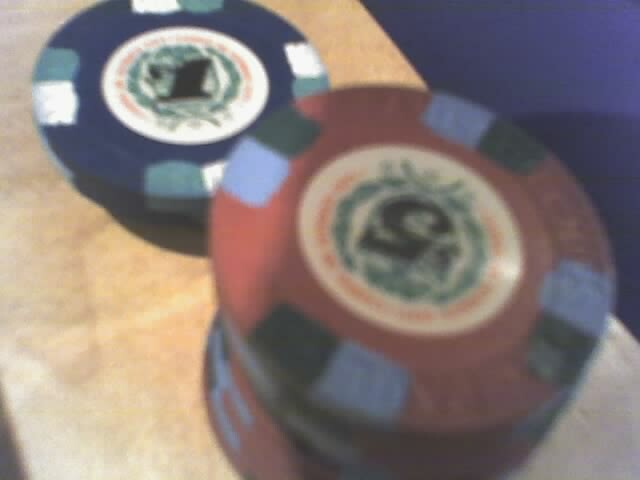This is a close-up, low-quality and blurred image of a collection of poker chips on a wooden surface. The wood appears to be light-colored, set against a dark blue background that might be a floor. Prominently, there are two stacks of circular poker chips. The left stack, containing blue chips, is shorter with about two chips. These blue chips feature light blue and white stripes on their outer edges and a white label in the center with a greenish-blue design and the black number one. The taller stack consists of red poker chips, approximately six or seven, positioned closer in the lower right. These red chips have light blue and black checks on their rims, with a light-colored center label showcasing a dark green emblem and the number five in black. The labels on the chips possibly have additional unreadable writing, potentially marking a casino name.